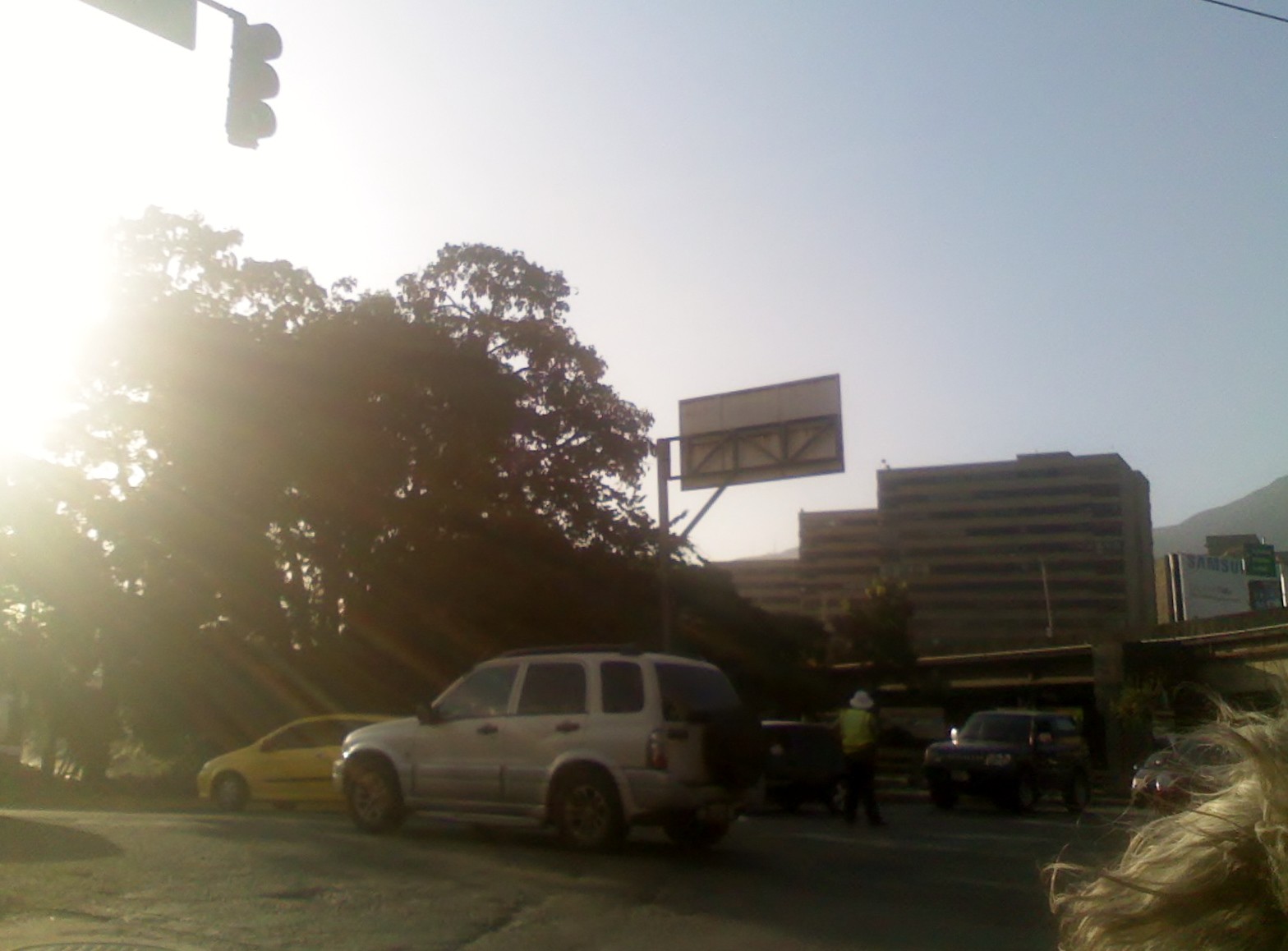The photograph captures a moment at a traffic light during late sunset. The descending sun casts golden rays on the scene, giving a warm hue to the small grayish SUV and the yellow sedan waiting at the light. Silhouettes of trees against the sky contribute to the tranquil atmosphere. In the upper left corner, the outline of a traffic light appears dark and indistinct, blending into the evening light. A street sign and an office building are visible in the background, along with the hazy outline of a distant mountain. In the right corner of the image, the wind lifts the blond hair of someone partially in frame. Nearby, a man in a white hat and a yellow sleeveless tank top is kneeling on the sidewalk, possibly a panhandler seeking assistance. The combination of these elements creates a vivid snapshot of urban life blending with nature at dusk.